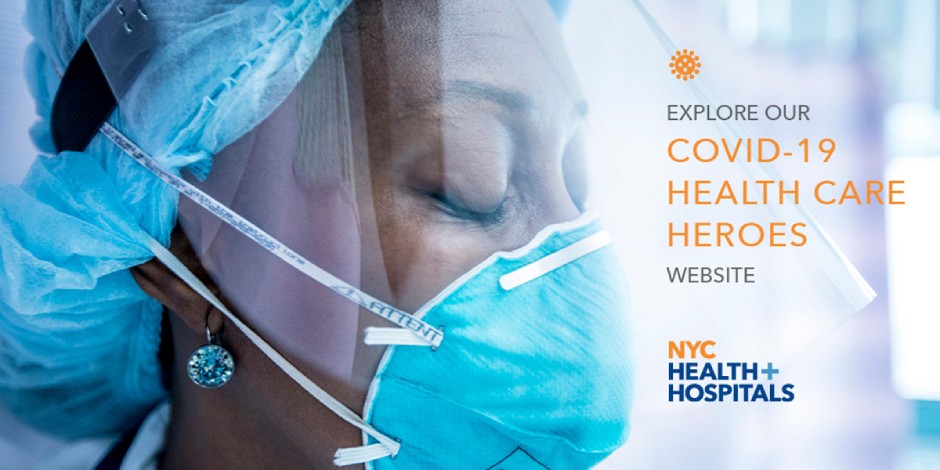The image depicts an advertisement or website excerpt with a close-up of an older Black woman. She appears to be in a hospital setting, indicated by her protective hairnet and mask. Her eyes are closed, and she is facing slightly to the right, approximately towards the 3:30 direction on a clock. She is wearing circular earrings with a silver outer rim and an aqua-colored center.

On the right side of the image, there is an icon of an orange sun. Below the sun, in black capital letters, it says "EXPLORE," followed by "COVID-19," "HEALTHCARE HEROES" in large orange font. Below that, in smaller black font, it says "website."

At the very bottom, in orange capital letters, it reads "NYC," followed by "HEALTH" in dark blue, "PLUS" in light blue, and "HOSPITALS" in dark blue, all in capital letters.

The entire image appears to have a glare or reflection, as if it is a photograph of a reflective surface, slightly obscuring the right 75% of the image.